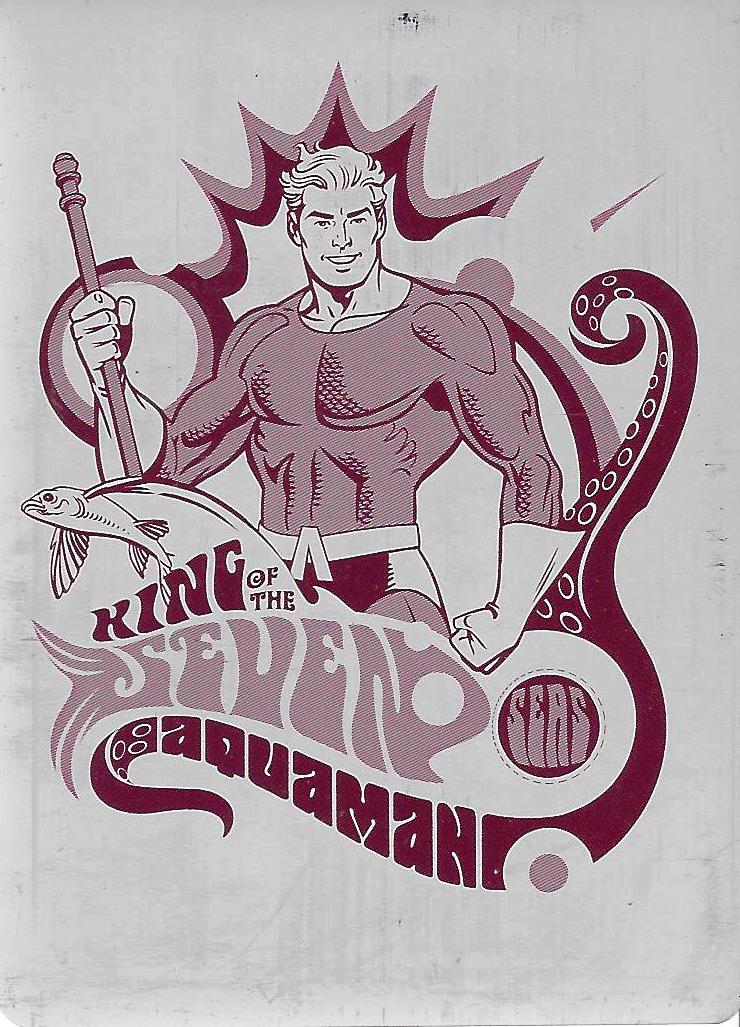This two-tone cartoon image of Aquaman features various shades of lighter and darker red. Aquaman, depicted with blonde hair and a muscular build, is smiling confidently. He is wearing a skin-tight suit and has a gauntleted left hand fisted at his side and his right arm raised, holding a trident. A starburst halo radiates behind his head, while stylized tentacles from an octopus frame the border on the bottom and right side of the image. A fish appears to be jumping above the word "King," which is part of the phrase "King of the Seven" written across the bottom. Below this, the name "Aquaman" is also written on the tentacle.